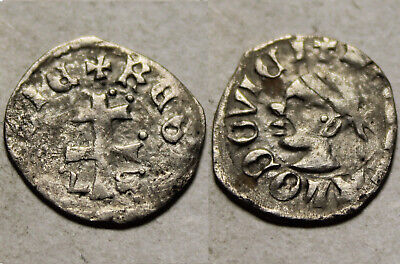This image presents a two-part view of an ancient, handcrafted coin against a light gray and tan stone-like background. The coin, exhibiting an irregular, rough, and unsymmetrical round shape, appears in both its obverse and reverse sides. The obverse (or head side) displays a profile of a figure facing left, adorned with a bandana, and is encircled by non-English text that arcs almost completely around the coin's edge. The reverse (or tail side) features a prominent double cross, consisting of one vertical and two horizontal lines, with additional foreign script written in an arc at the top. The coin's surface shows signs of age and discoloration, with hues of silver and dark brown-black patches, reflecting its historical authenticity and rich patina.